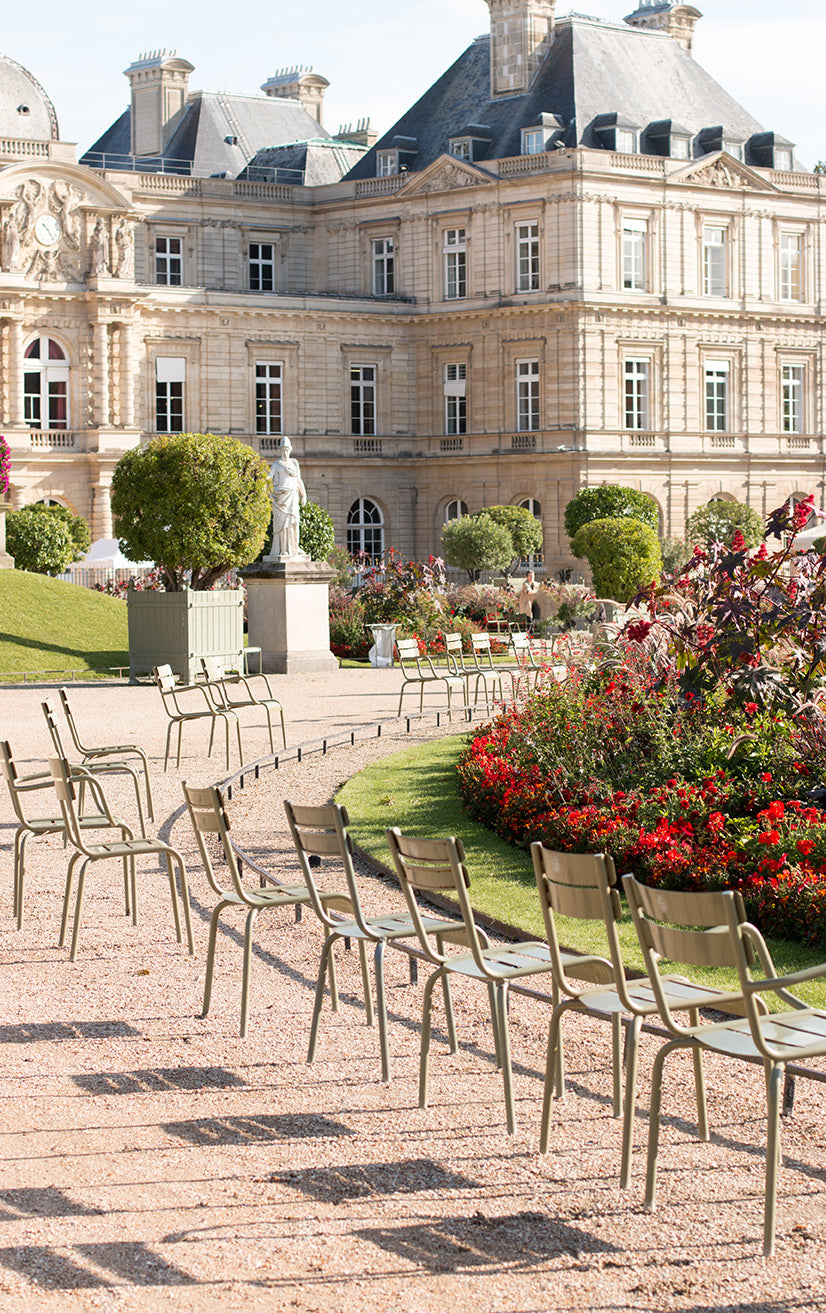This highly detailed color photograph, in portrait orientation, captures the ornate exterior of a large mansion reminiscent of the Versailles palace. The mansion is constructed with light-colored stone and features three definitive stories, with additional windows protruding from the roof, suggesting a potential fourth attic-like level. The mansion's facade is adorned with numerous chimneys and windows, showcasing its intricate and grand design.

In the foreground, a curving gravel path made of small stones leads the viewer's eye through the image, initially veering to the left before centering again. The path is surrounded by a meticulously curated garden area populated with vivid red and green flowering bushes, neatly manicured grass, and round, carved bushes. A pedestal supports a fancy statue, likely made of marble, further accentuating the garden's opulence.

Adjacent to the gravel path, a collection of silver metal chairs is arranged in an arc, their backs facing outward toward a low-level banister that acts as a boundary for this elegant courtyard. These chairs are strategically placed to face the garden, with sunlight streaming from the right side of the image, casting a warm glow over the scene.

Overall, the interplay of the grand architectural backdrop, the stately garden, and the orderly arrangement of chairs offers a picturesque and inviting outdoor setting.